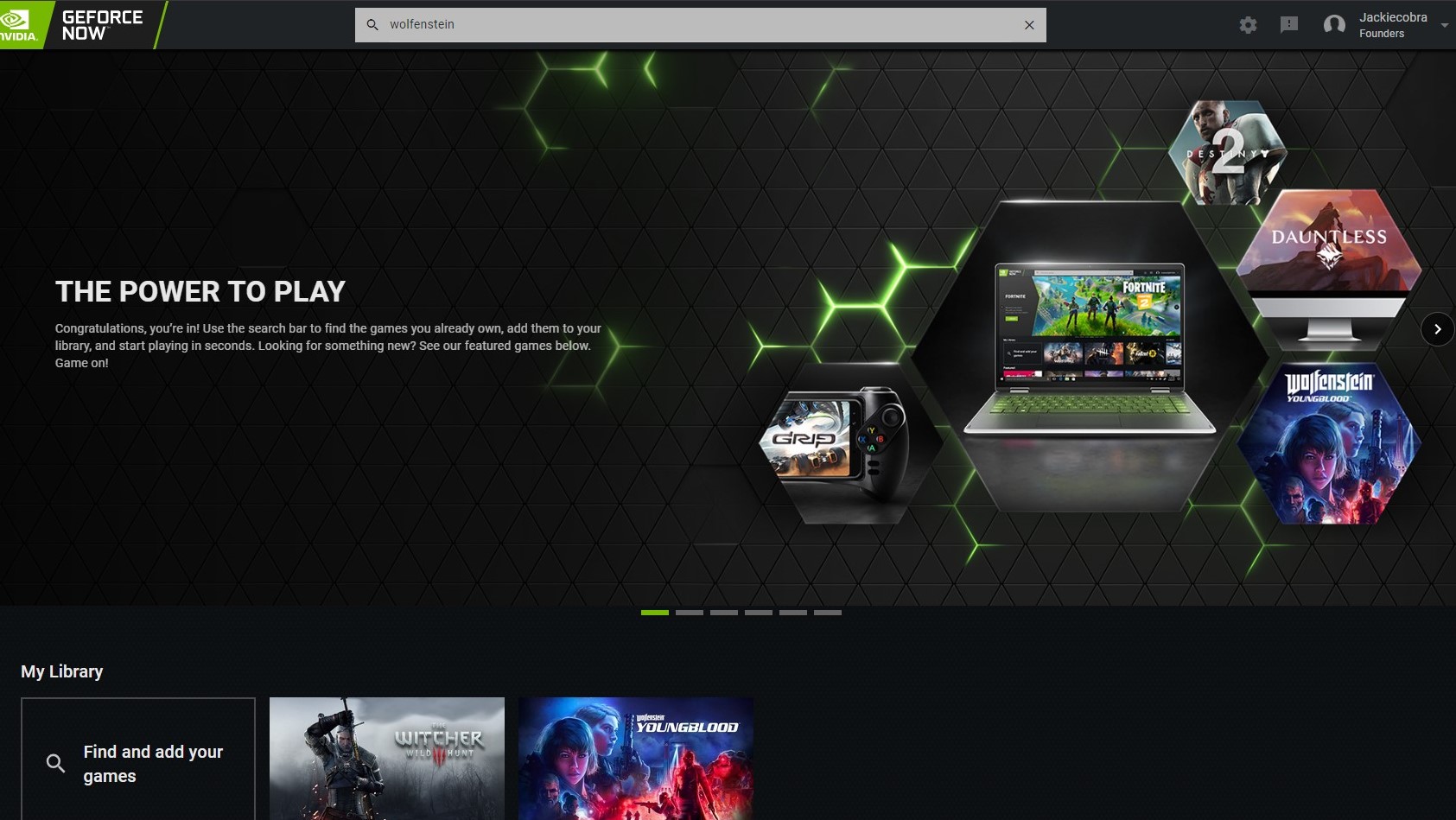In the upper left corner of the image, there's a green square with white text that appears to be partially cut off, but it likely says "NVIDIA." Adjacent to it, "GeForce NOW" is clearly visible. Centrally, there's a gray search bar containing the black text "Wolfenstein," with a small 'X' icon on the right for clearing the search term. On the far right, a series of icons are lined up, including a settings gear, an exclamation point, what appears to be a headphone icon, and an account name "Jackie Cobra" with a dropdown labeled "Founder."

Below, a prominent banner reads, "The Power to Play! Congratulations, you're in! Use the search bar to find the games you already own, add them to your library, and start playing in seconds. Looking for something new? See our featured games below." To the right of this text, an open laptop displays the game Fortnite in play, and there's a gaming controller labeled "Grip."

Underneath, a selection of featured games includes titles such as Destiny 2, Dauntless, and Wolfenstein: Youngblood. Further down on the left, under a section titled "My Library," users are instructed to "Find and add your games with the search icon." Below this instruction, a list of games includes "Witcher" and "Youngblood." 

This meticulously detailed caption provides a comprehensive overview of the visual elements in the image.